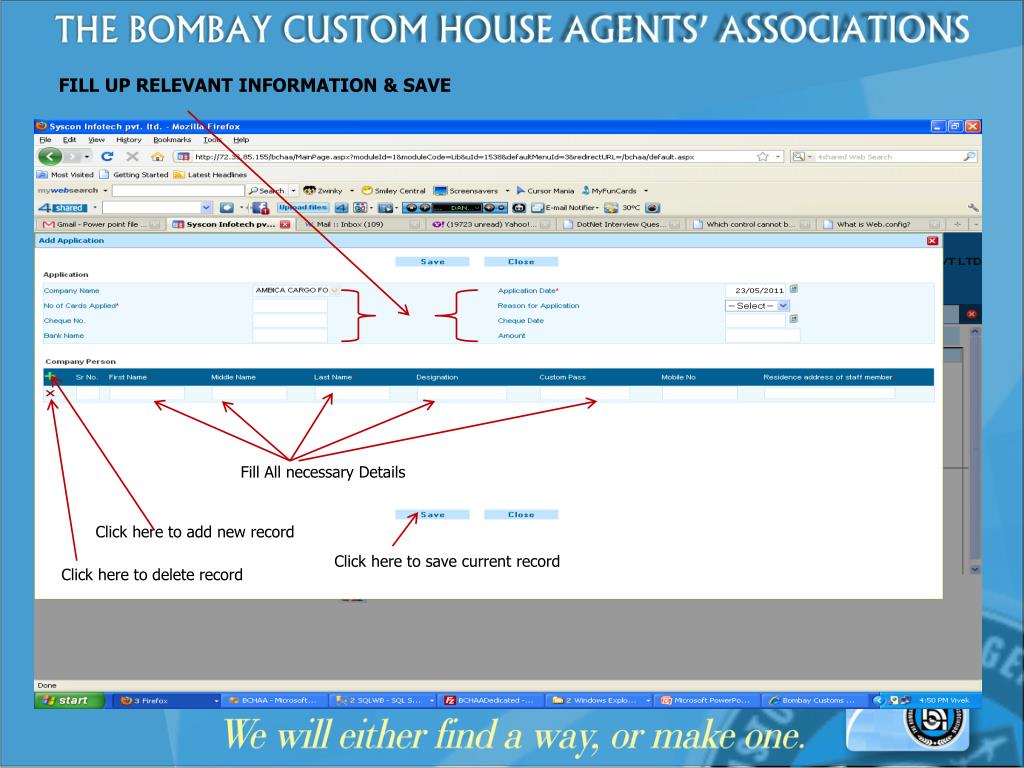This is a detailed screen capture from a computer, showcasing the instructions for completing a form on the Bombay Custom House Agents Associations' website. The background features a light blue hue, and at the top of the screen, in all-capital white font, it reads: "THE BOMBAY CUSTOM HOUSE AGENTS ASSOCIATIONS." Directly beneath this, in black capital letters, the text "FILL UP RELEVANT INFORMATION AND SAVE" is displayed.

The screenshot highlights various input fields with red lines and arrows, indicating the areas to be filled out. The fields include "Company Name," "Number of Cards," "Checkout Number," "Base Name," "Application Date," "Change Date," and "About." However, the small print makes it difficult to read the details clearly.

Below these fields, there is a taskbar featuring multiple options, which are also too small to read clearly. Red arrows point to each box with the instruction "FILL ALL NECESSARY DETAILS."

Further instructions are provided:
- "Click here to add new record," with an arrow pointing to the relevant button.
- "Click here to delete record," indicating the button for deletion.
- "Click here to save current record," with an arrow pointing towards the Save button.

Next to the Save button, there is a blue Close button. Observably, the screen capture is from a Microsoft computer, as indicated by the numerous tabs (nine in total) open at the bottom of the screen.